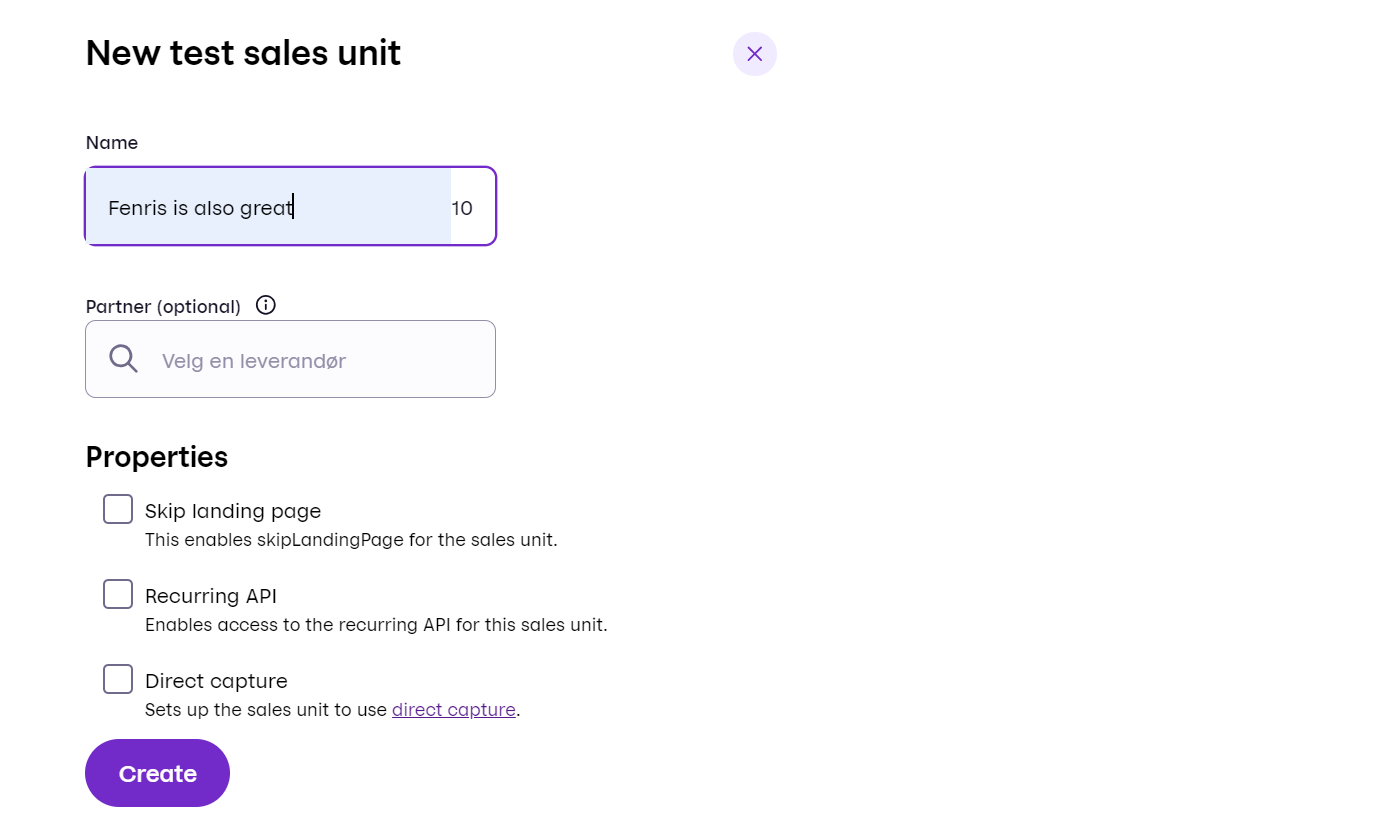An image of a website form featuring a clean white background dominates the scene. In the top left corner of the form, bold text reads "New Test Sales Unit." On the far right-hand side sits a light purple button adorned with a deep purple 'X,' indicating a close function.

On the left side of the form, a small label specifies "NAME" in uppercase letters. Directly beneath this label is a text box with a distinct purple border. The majority of the text box is filled with a blue hue, with a small white segment on its right side. Inside the blue section, the phrase "Fenris is also great" is typed out. A blinking cursor indicates the current input location within the box. In the white segment, the number "10" is visible, possibly denoting the length or another metric related to the text.

Further down, another label reads "Partner" accompanied by the word "optional" in parentheses. Adjacent to this label is a small circle containing the letter "I," likely an information tooltip. A second text box is positioned below, featuring a magnifying glass icon on the left, hinting at a search functionality. Alongside this icon, text reads "VELC and LEVR and DOR," suggesting placeholders or example text in another language.

Moving towards the left side of the form, a heading labeled "Property" appears. Below this heading, three unchecked checkboxes are arranged vertically, each paired with a description:
- The first checkbox is labeled "Skip Landing Page." A smaller, descriptive text beneath it notes, "This enables skip landing page for the sales unit."
- The second checkbox, marked "Reoccurring API," includes the note, "Enables access to the reoccurring API for the sales unit."
- The final checkbox is titled "Direct Capture." The descriptive text underneath explains, "Set up the sales unit to use direct capture," with the term "direct capture" underlined and colored in purple, suggesting it is a clickable link.

At the bottom left corner of this section, a prominently displayed purple button with rounded edges reads "Create" in white text, inviting the user to submit or finalize the form.